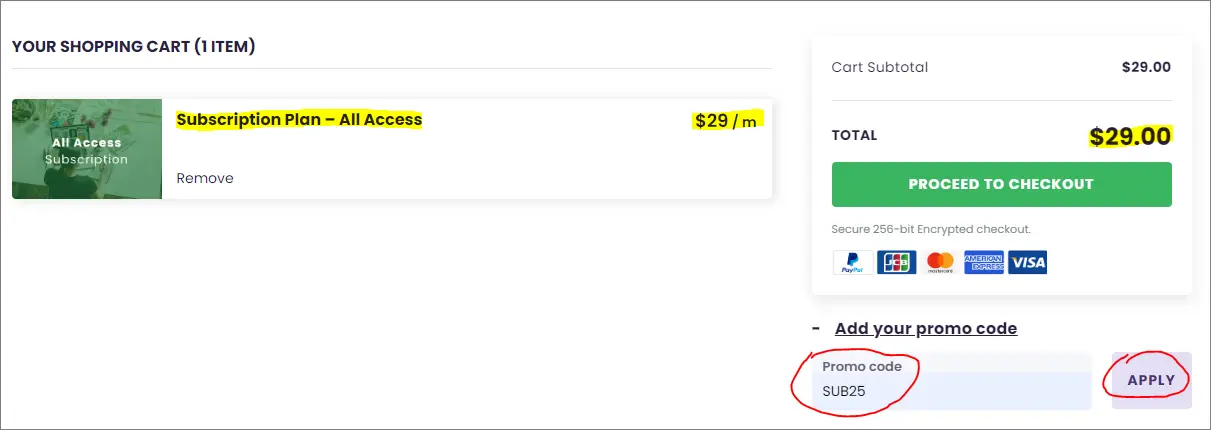A screenshot of a computer screen displaying an online shopping cart. At the top of the screen, the header reads "Your Shopping Cart" in bold black text, followed by "(1 item)" in parentheses. Below, a green-highlighted section shows "All Access Subscription" along with some small, indistinct images. 

Further down, a yellow-highlighted box details the subscription plan, labeled "All Access," priced at "$29/month." There is an option to remove the item next to it. To the right, the cart subtotal is displayed as "$29." This amount is repeated in the total section beneath it, confirming that the total cost is also "$29."

Towards the bottom of the screen, there is an option to add a promo code. The field for entering the promo code and the "Apply" button are both circled in red marker, emphasizing their importance. A "Proceed to Checkout" button is prominently displayed for finalizing the purchase.